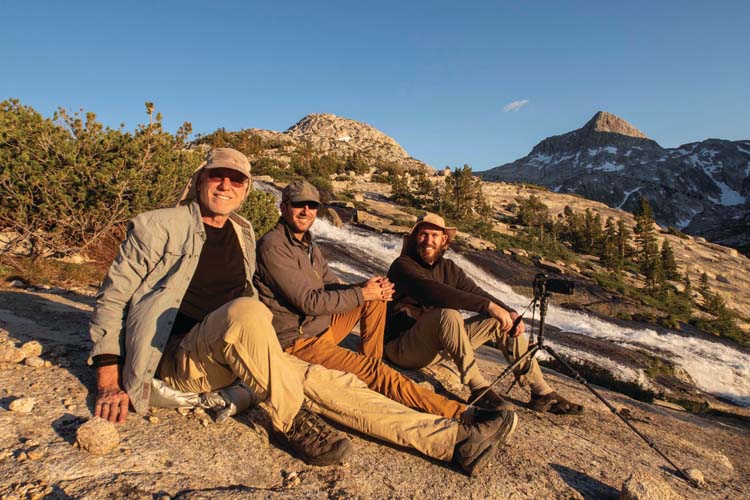In this outdoor image, a trio of men is seated on a rocky outcrop on the side of a mountain enshrouded by a natural landscape. They are outfitted in similar warm attire, but each man sports different colors and styles. The man on the left is clad in a white jacket over a black undershirt, wearing pale beige slacks and a snug hat. The middle figure, dressed in a gray parka with dark beige slacks, also wears a ball cap and is distinguished by his seated position on dirt terrain of about a 30-40% grade. The third man on the right dons a cowboy hat and a black jacket, paired with pale beige slacks and, like the others, black shoes. 

A noticeable feature in the foreground is a camera set up on a tripod, suggesting they are engaged in some form of photography. Dominating the upper quarter of the frame, the clear blue sky stretches above the peaks. The backdrop features scattered trees and patches of snow, which create a picturesque landscape. Amidst this rugged terrain, a query arises whether the visible streaks are flowing water or lingering snow, amplifying the scene's complexity. The mountains in the distance display a mix of snow and rugged rock, adding a serene yet raw beauty to the image.